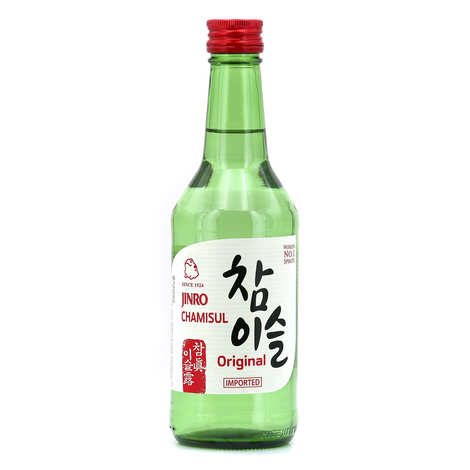This is a high-quality image of a clear green glass bottle, approximately eight inches tall and tapering up to a red aluminum screw cap at the top. The bottle, which is likely around 12 ounces, is filled with clear liquid, leaving a small air gap at the top. The front of the bottle features an intricate label with a white background. In the center of the label, there are black Chinese characters, below which it reads "Jinro Chamisu Original" in English. The word "Imported" is prominently displayed in red letters, enclosed within a square. To the left of this central text, a section of the label has a red background with additional white Chinese lettering, and above this is more text that is difficult to decipher. The overall design suggests that this might be a bottle of Japanese sake or a similar alcoholic beverage. The label's shape is distinct with an offset square design that includes two pointed ends, adding to the sophisticated appearance of the bottle. The classic green glass and red cap combination enhance its aesthetic and high-quality feel.